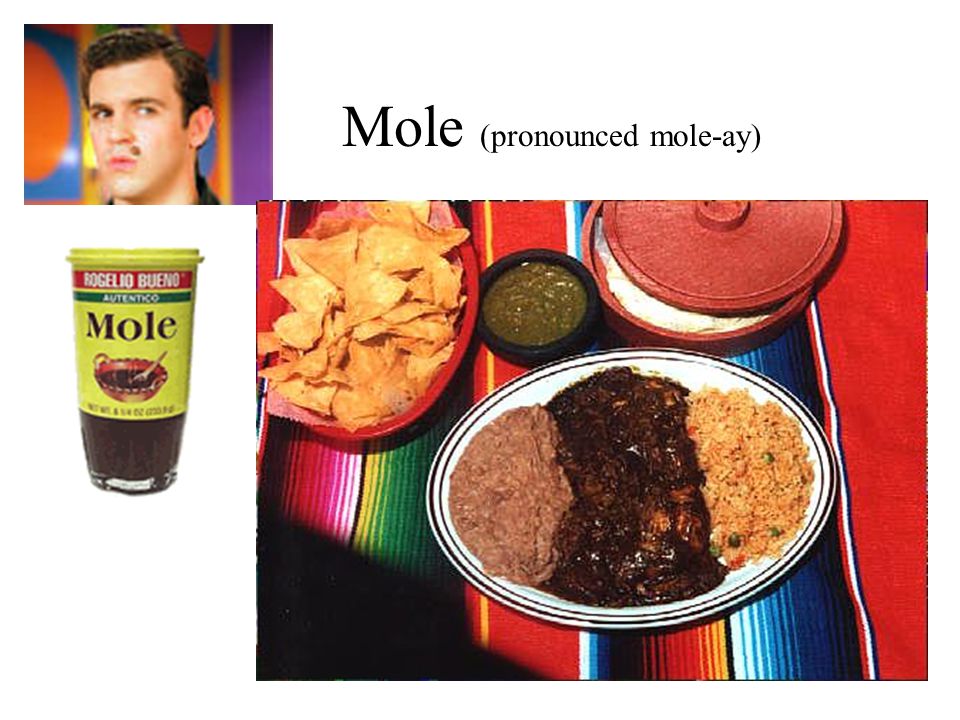The image is a vivid and informative composition featuring multiple elements centered around mole sauce. In the upper left, there is a small color photograph of a man, specifically the actor Fred Savage, with a facial mole. Savage is looking suspiciously to his left, set against a brightly colored background. Below this image, there is a jar with a bright yellow label featuring the word "mole." On the bottom left of the image, this jar represents mole sauce, showcasing what it would look like if purchased. Dominating the bottom right portion is the largest photograph, capturing a view of a Mexican meal laid out on a colorful, striped Mexican tablecloth. The meal includes a plate with beans on the left, rice on the right, and enchiladas with dark, mole sauce in the center. Accompanying the plate are a black container of green salsa, a red basket of tortilla chips, and a ceramic tortilla container with a lid that is slightly open. In the top right corner of the image, set against a white background with black text, is the word "mole," along with its pronunciation in parentheses "M-O-L-E-A-Y." This image merges photographic realism with graphic design and typography to convey detailed information about mole sauce.